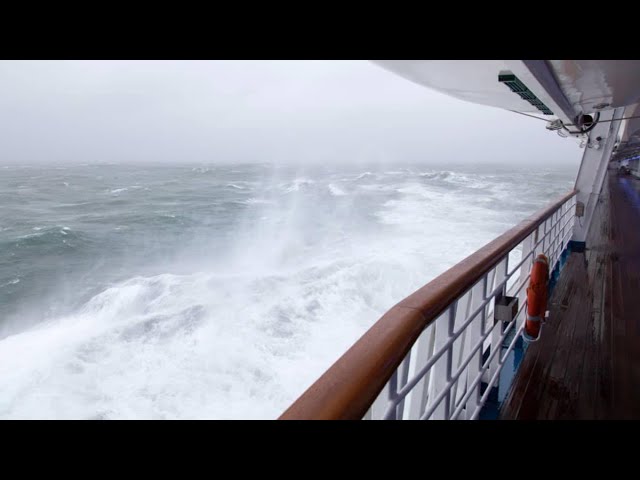This photograph, taken from the deck of a white ship or yacht with brown railings and a wooden deck, captures a dramatic scene of marine life during a storm. The image showcases a greyish, turbulent sea with rough, white-capped waves. The stormy seas and the serene, overcast grey sky create a stark contrast. The photo includes an orange life preserver hanging on the rails and a red lifeboat tube on the deck, which appears shiny and slick, likely due to mist from the crashing waves. Despite some motion blur and low resolution, contributing to the slightly compressed and blurry appearance, the details of the rocky, stormy ocean to the left and the upper deck structures above are discernible. Black bars at the top and bottom of the image suggest it may have been taken from a video. The overall atmosphere is one of rugged marine adventure, with the violent storm pushing the ship in various directions amidst a backdrop of tumultuous waves and a somber sky.